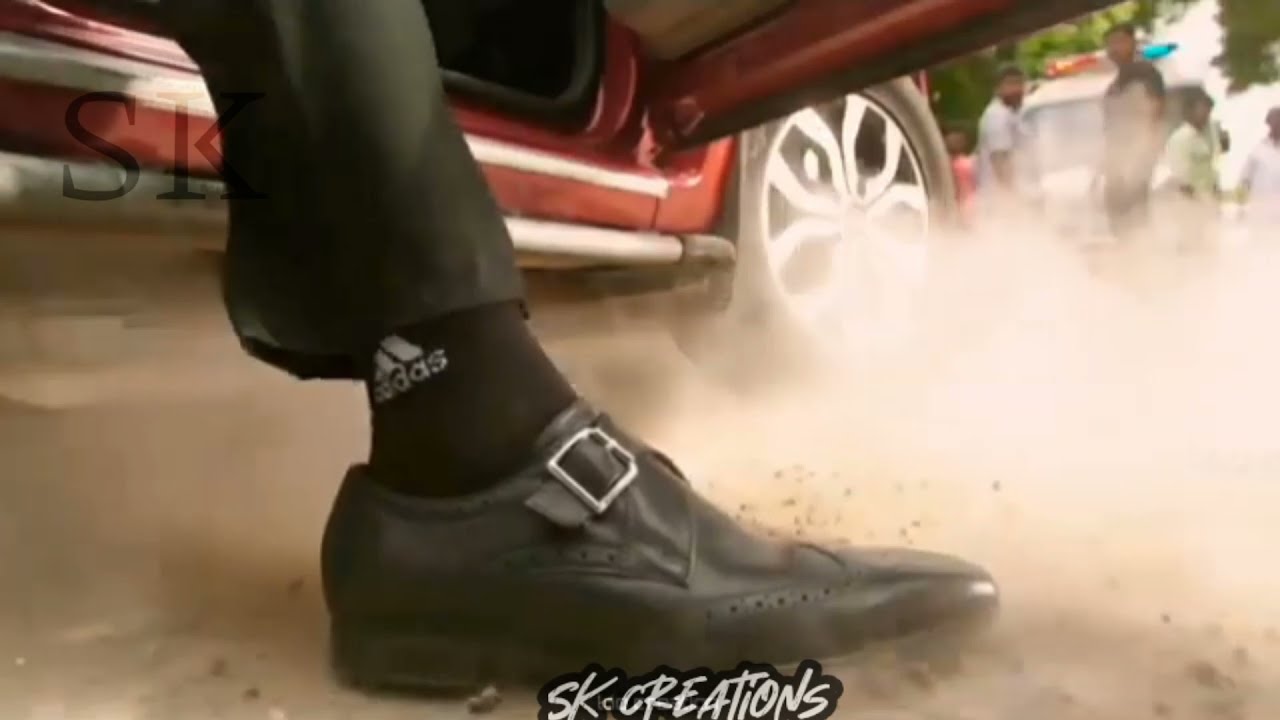A close-up image depicts a man stepping out of the passenger door of a red sports car onto a dusty dirt road. The focus is on the man's right leg, captured from just below the knee down to his black dress shoe, which features a silver buckle near the top. He is dressed in black slacks and black Adidas socks with the distinctive white logo. The impact of his foot on the ground has kicked up dust and small rocks around him, adding a dynamic sense of movement. In the background, several people, who appear to be Indian, are intently watching the scene unfold. Among them, an emergency vehicle with police lights is visible, further hinting at the significance of the moment. The image also includes the text "SK Creations" at the bottom.